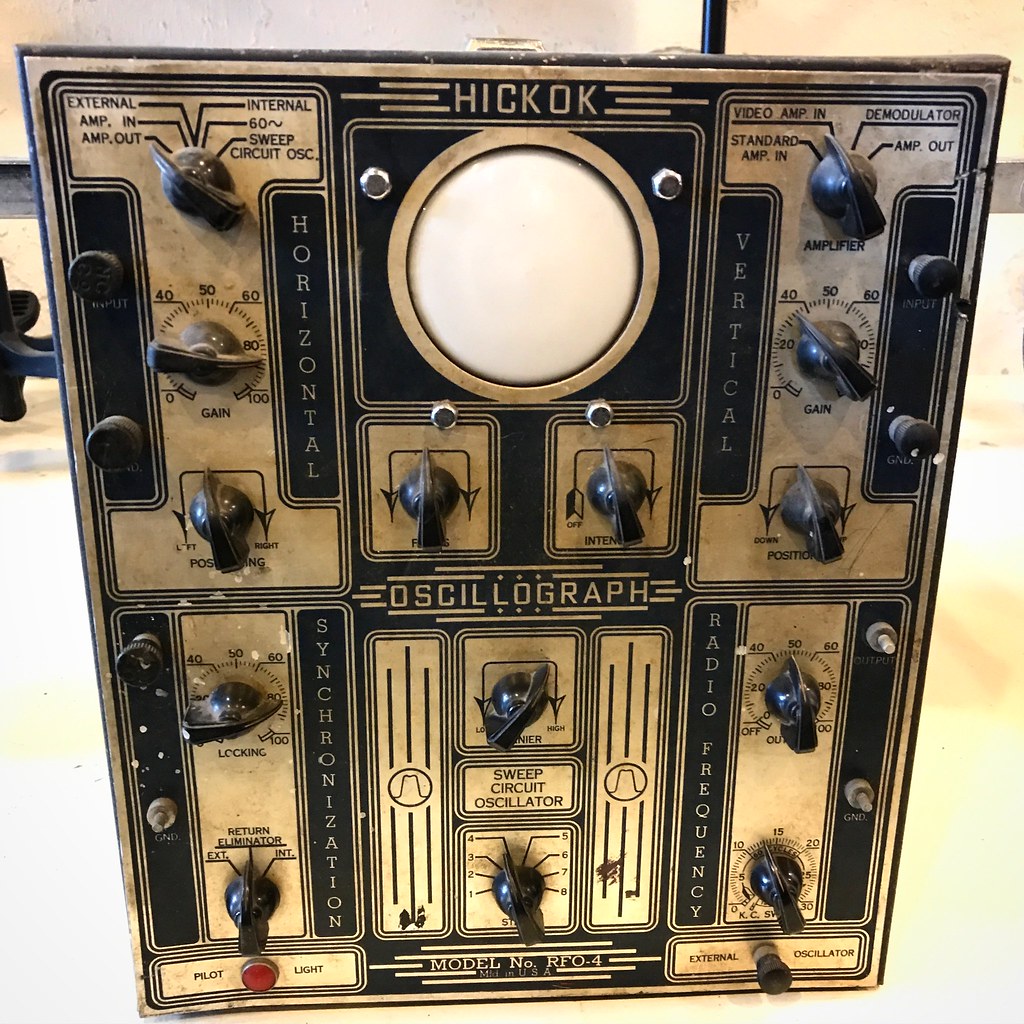This image features a tall, rectangular control board with a blend of vintage and complex electronic components, likely from an old radio station or similar setup. The control board is mounted against an off-white wall and comprises a gray silvery metal frame with both tan and black backgrounds. At the very top of the board is inscribed "Hickok model number RFO4" in silver letters, indicating the manufacturer. 

Positioned centrally at the top is a prominent pilot light, which is red and white. Surrounding this light are several groups of knobs and dials arranged symmetrically: three knobs on the top left, and three knobs on the top right. Below these, there are columns of knobs and switches with distinct labels. Directly beneath the pilot light is a section with two horizontally aligned knobs, labeled "oscillograph" and "sweep circuit oscillator". To their right and left are additional vertical columns of two knobs each, labeled with terms like "radio frequency" and "synchronization". 

The control board's structure is compartmentalized with distinct sections, each featuring silver on black lettering indicating functions like "horizontal" and "vertical". The overall composition is dominated by these electronic components, reflecting an era of intricate analog technology.